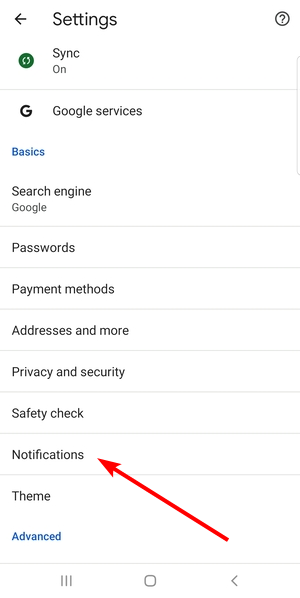This image appears to be a screenshot from a mobile phone displaying a settings page. The background is white with black text, separated by thin gray lines. At the bottom, there are three navigation icons: three vertical bars, a square with rounded edges, and a back arrow, all in gray. 

At the top of the screen, the word "Settings" is displayed in black, accompanied by a back arrow on the left and a question mark icon on the right. Below that, the text "Sync on" is shown with a small green circle featuring a white checkmark.

The next section is titled "Google Services" and begins with a black "G". Below this title, various options are listed:

- **Basics** written in blue
- **Search engine:** Listed as Google
- **Passwords:** No information displayed
- **Payment methods:** No information displayed
- **Addresses and more:** No information displayed
- **Privacy and security:** No information displayed
- **Safety check:** No information displayed
- **Notifications:** Marked with a superimposed red arrow pointing from above the rightmost phone icon towards this section
- **Team:** No information displayed

At the bottom, the text "Advanced" is shown in blue. There are thin horizontal lines that divide each of these sections for clarity. Additionally, a tiny vertical black line is visible to the right of the "Sync on" and "Google Services" area.